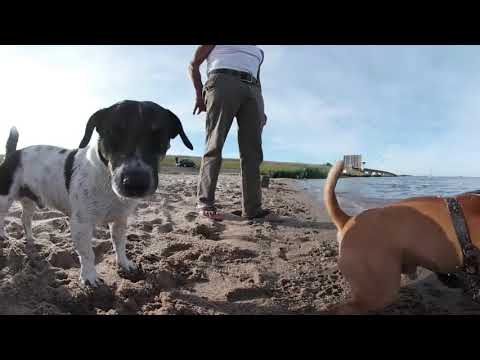The photograph captures an intimate, outdoor moment at the beach featuring two small dogs and a standing figure, presumably of their owner whose upper body is not visible. The dog on the left is smaller, black and white, with a black head, white muzzle, and a black stripe on its back, standing on the tan, footprint-covered sand and looking directly into the camera. On the right, a tan dog partially visible from the shoulders back, with a lifted tail, stands near the bluish shoreline; its harness hints at its readiness for a beach adventure. Between the dogs, the figure wearing tan pants, a dark brown belt, and a white sleeveless shirt stands upright, facing the right. The backdrop features a lush green land, a distant white building on the coastline, and a cloudy sky, encapsulating the serene, cloudy beach day.